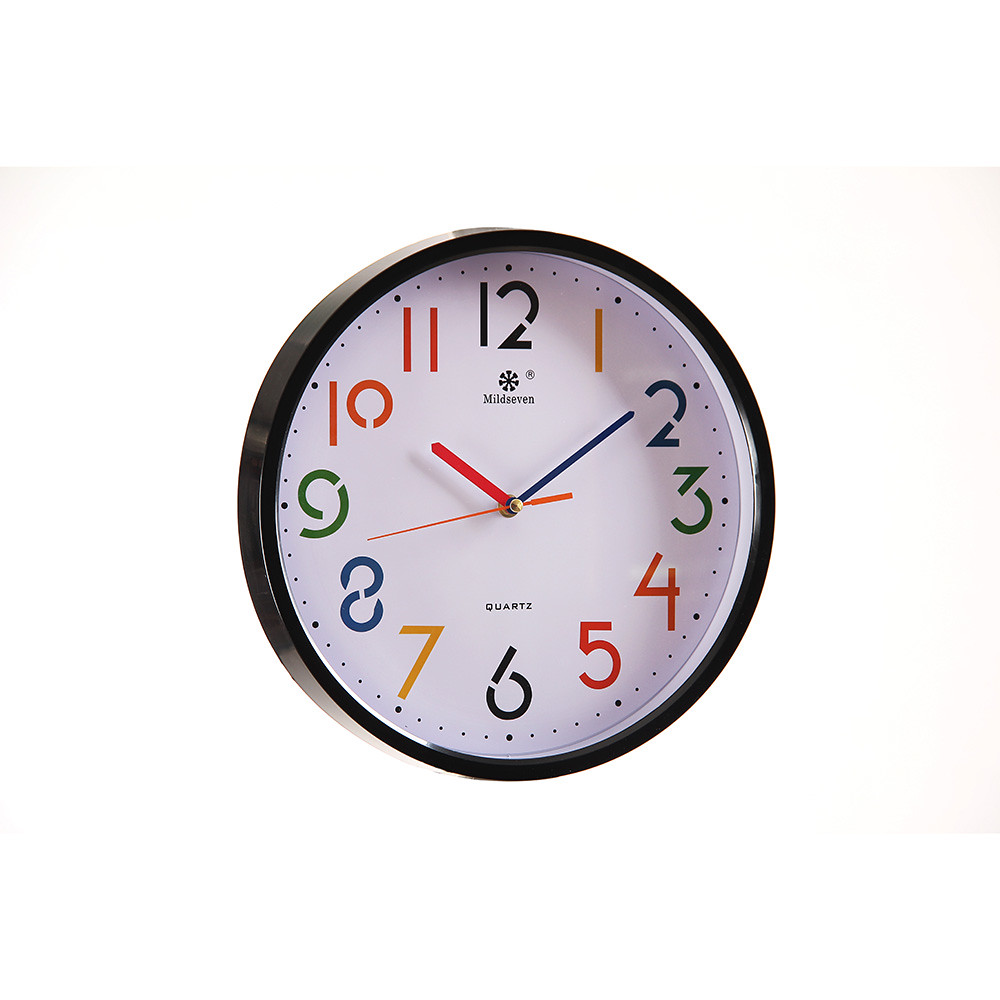This image features a hanging wall clock against a predominantly white background with subtle gradients. The top corners showcase a slight gradient, while the bottom right corner transitions from white to an off-white or cream hue. The bottom left remains pure white, blending seamlessly with the central portion of the background.

The clock itself is encased in what appears to be a black plastic housing, with a clear protective panel covering its face. The clock face is white, prominently displaying the brand name "MILD 7" and the word "QUARTS" in bold black letters. The numerals are rendered in both black and red, adding a touch of color contrast. The hour hand is red, the minute hand is black, and the second hand is also red, providing a cohesive yet visually engaging design.